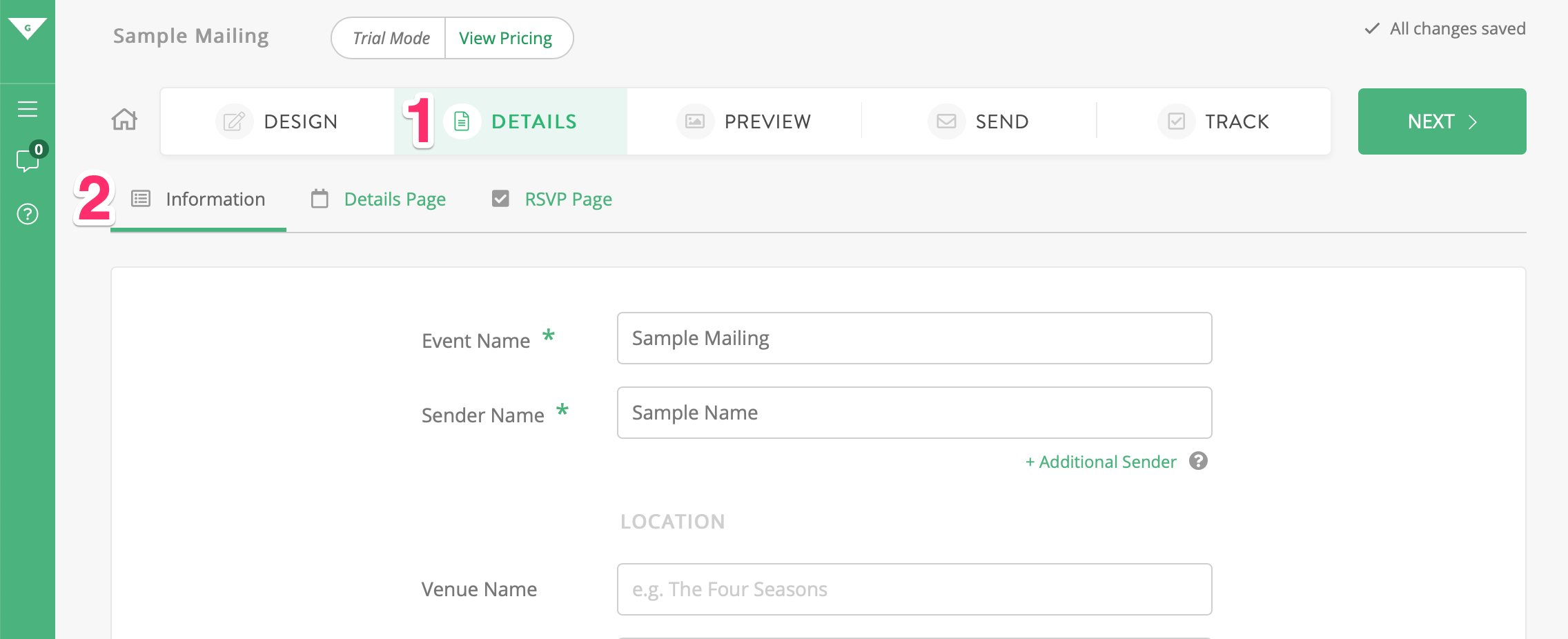This image captures a computer screen displaying a sample mailing interface. The screen's background is gray, with several elements highlighted in green for emphasis. A skinny green rectangle extends vertically along the left-hand side, contributing to the visual structure. 

At the top of the interface, the words "Sample Mailing" are prominently displayed, flanked by the options "Trial Mode" and "View Pricing." Below this header, a horizontal navigation bar presents various stages of the mailing process: "Design," "Details," "Preview," "Send," and "Track." In the top right-hand corner, a clickable "Next" button is visible, encouraging the user to proceed to the next step.

A red, white-lined number "1" is positioned next to the "Details" button, indicating a point of focus or step in the process. Further down and slightly to the left, a red number "2" appears near the "Information" section, guiding the user to another critical area. The "Details" and "RSVP" pages within this section are highlighted in green, denoting their current active status or importance.

The combination of these visual cues and labeled sections provides a clear, navigable interface for users engaged in the mailing process.